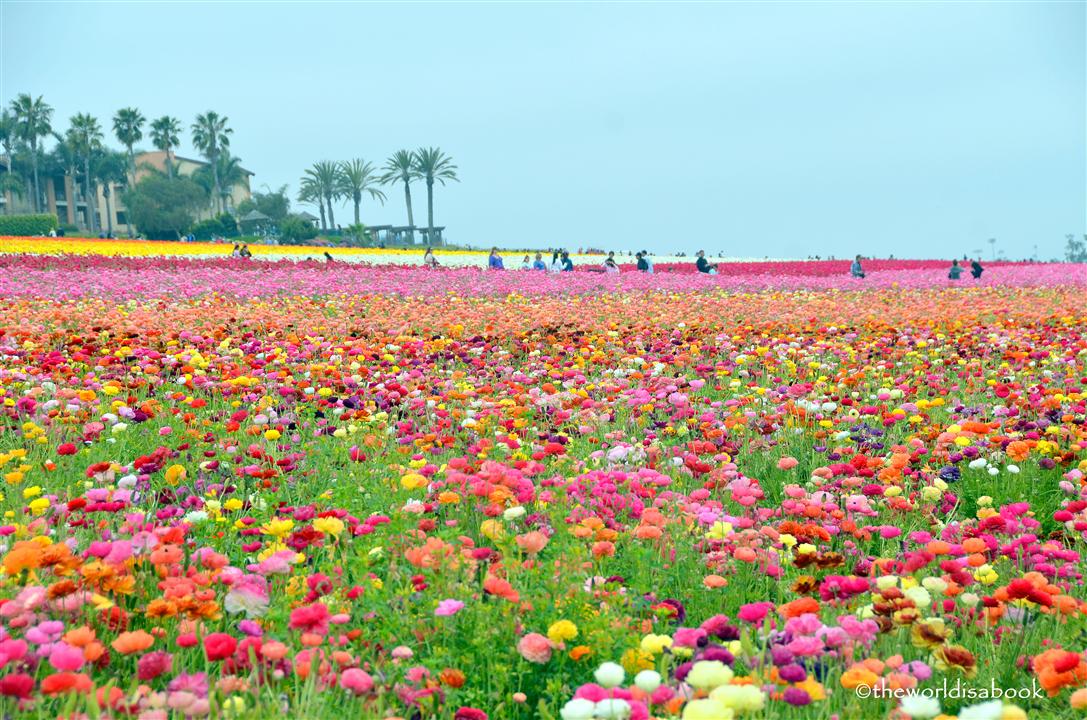The photograph captures a vast field dominated by pink and red flowers, interspersed with splashes of orange and yellow hues, creating a vibrant and colorful landscape. Amidst the flowers and patches of grass, several birds and people can be seen moving through the middle and back sections of the field, enjoying the picturesque scenery. In the background, a house or small hotel with surrounding palm trees is located in the upper left corner of the image, adding to the idyllic atmosphere. The sky overhead is a soft mix of blue and white, contributing to the serene setting. The bottom right corner features a copyright notice that reads "the world is a book," written in white.